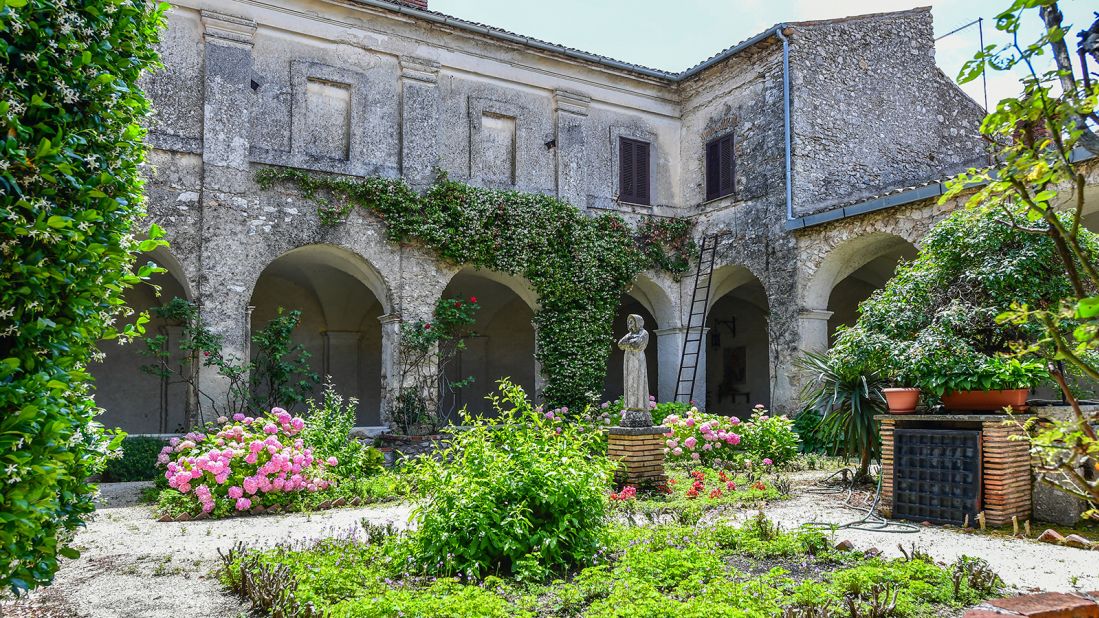The photograph depicts an old, multi-story building with a weathered rock and stucco facade, indicative of its age and lack of recent habitation. Mildew stains surround the windows, some of which are sealed shut, while others remain open or adorned by a ladder. The structure features large pillars, one of which is entwined with ivy reaching up to the second floor. The building's courtyard is a blend of stone and cobblestone, with an outdoor fireplace and numerous unkempt plants, including tall bushes, shrubs, and weeds. Amongst the vegetation are two beautiful bushes with large pink blossoms and what may be tulips. Central to this scene is a statue of a woman in a long dress, possibly the Madonna, standing with crossed arms on a blond brick pedestal. Despite the courtyard's overgrown state, it receives ample natural light, enhancing the vivid greenery and blue sky with scattered clouds in the backdrop. This courtyard, though neglected, retains an inherent charm and potential for restoration.